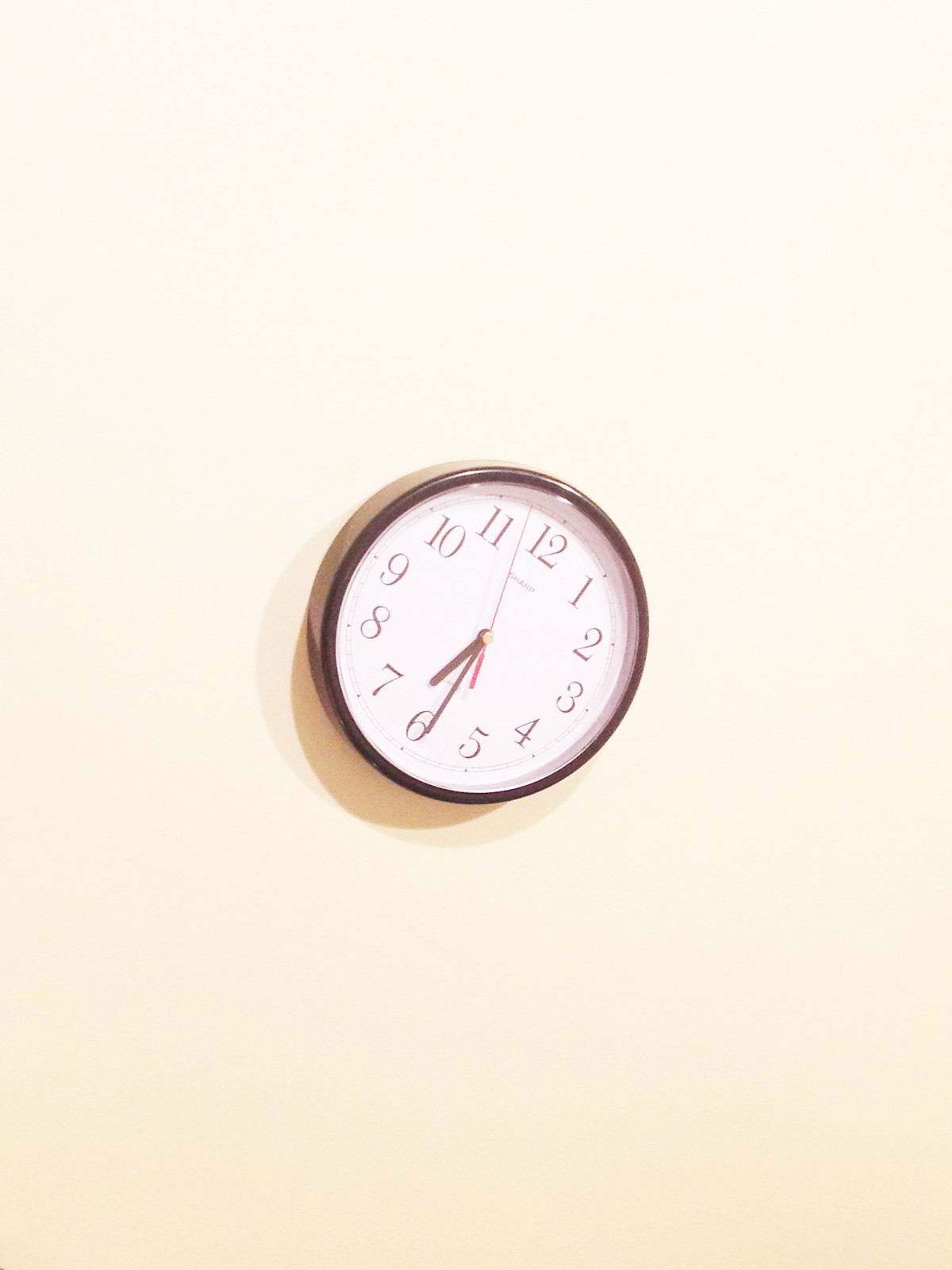This is a detailed portrait-oriented photo of a traditional round analog clock taken straight on, possibly mounted on a featureless, white wall. The background of the image is a light tan, slightly washed out in light. The clock itself has a black case with black hour and minute hands, black numbers, and a red second hand. The time displayed is 6:29 and 57 seconds. The clock is tilted slightly clockwise, causing the topmost digit to fall between the 10 and 11 positions rather than directly at 12. Despite the tilt, the photo captures the simplicity and stark contrast of the clock’s design against the plain background.